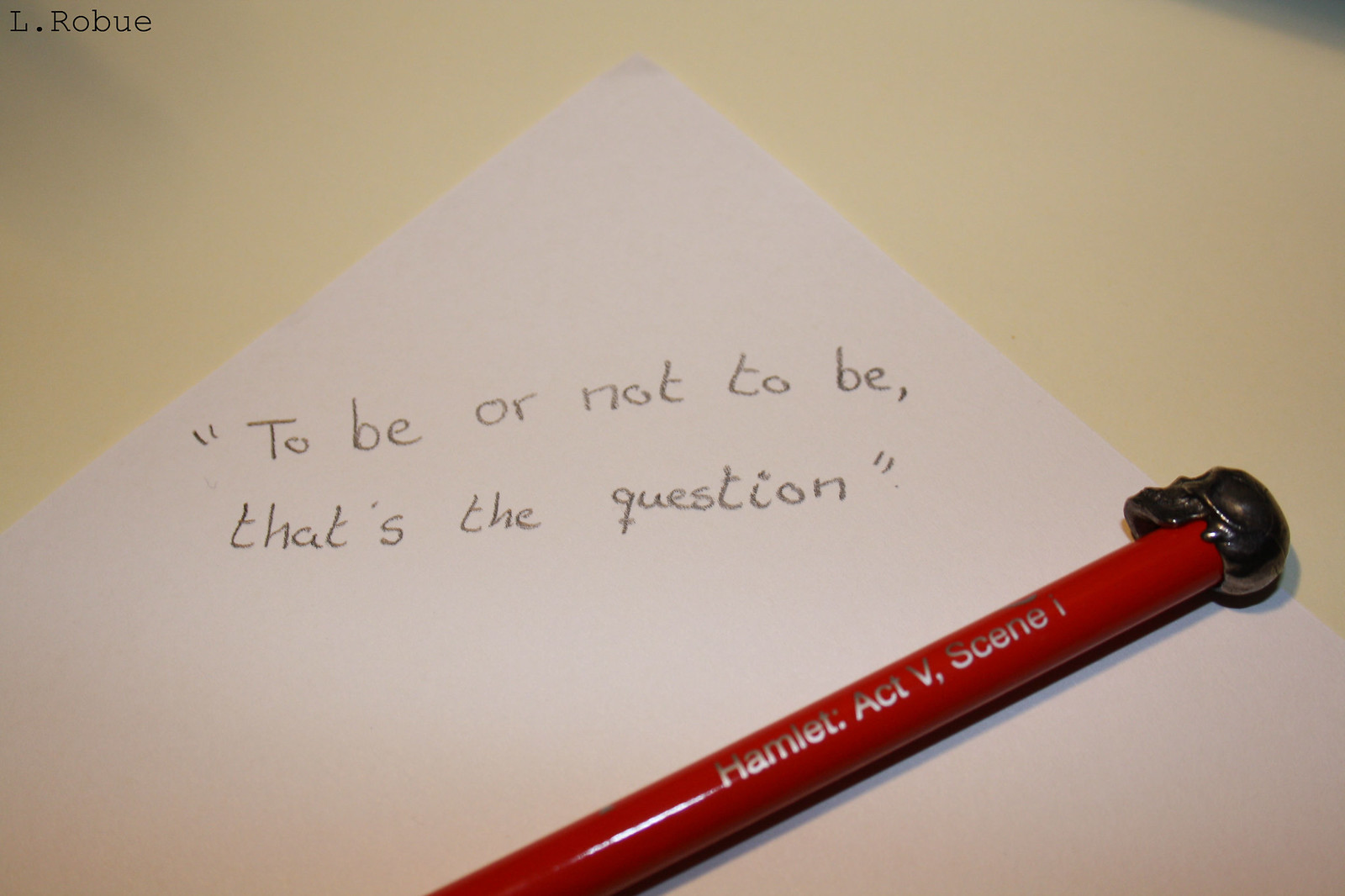This color photograph captures a white sheet of paper with a handwritten quote "To be or not to be, that's the question" in black ink. The paper is laid diagonally on a light beige or tan tabletop. At the top of the page, there is the text "L.ROBUE" in the upper left corner against the background. A bright red pen with a small black skull-shaped top rests on the lower right-hand corner of the paper, featuring the silver text "Hamlet, Act 5, Scene 1." The overall composition highlights the juxtaposition of the classic Shakespearean quote with the detailed thematic pen. The informal handwriting and the setting on the beige surface give the image an everyday, candid feel.